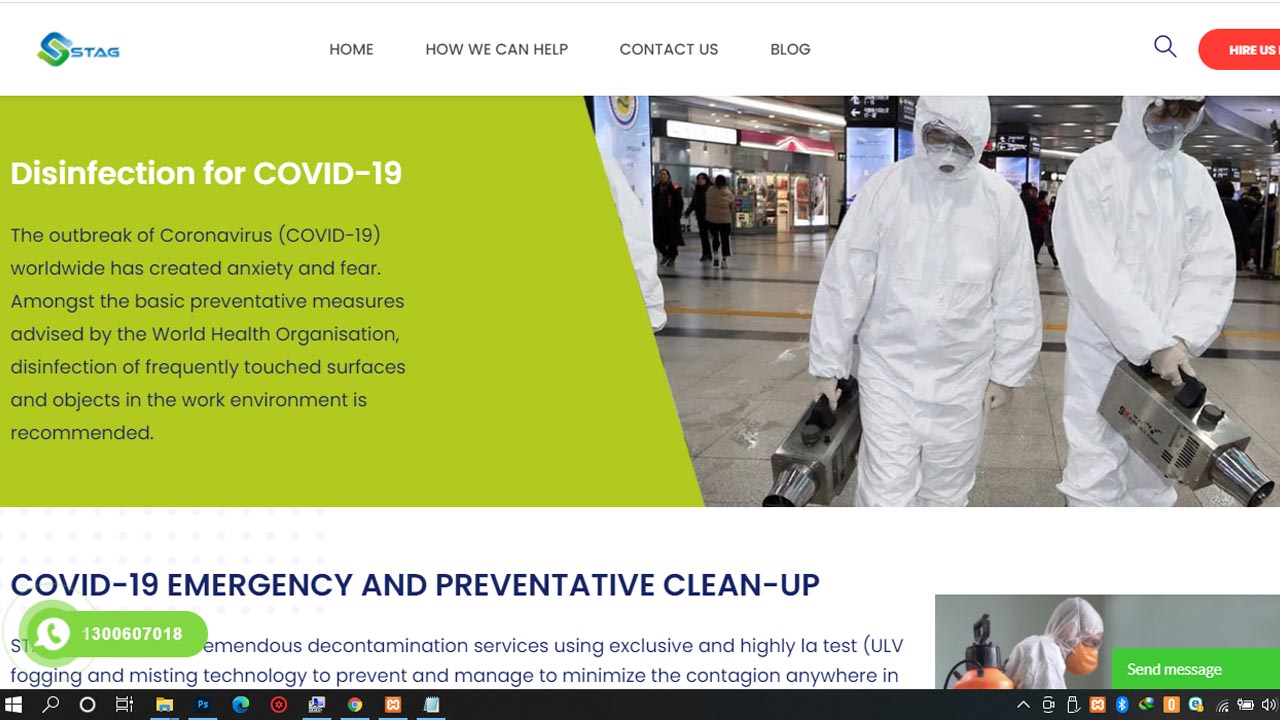The image depicts the landing page of a website called STAG. At the top, the navigation menu features links labeled as "Home," "How We Can Help," "Contact Us," and "Blog." To the left of this menu, there is a prominent "Hire Us" button. Below the header, a large banner reads: "Disinfection for COVID-19" and highlights the urgency brought about by the outbreak of the coronavirus (COVID-19) worldwide, mentioning the anxiety and fear it has sparked.

The banner text goes on to recommend the disinfection of frequently touched surfaces and objects within the work environment, as advised by the World Health Organization. Directly underneath, there's another message that reads: "COVID-19 Emergency and Preventive Cleanup," emphasizing their service focus. Additionally, a section displaying a contact number, "1-300-607-18," is visible, inviting users to get in touch for their services.

The image also includes visuals of individuals dressed in hazmat suits, reinforcing the seriousness and professionalism of STAG’s disinfection services.